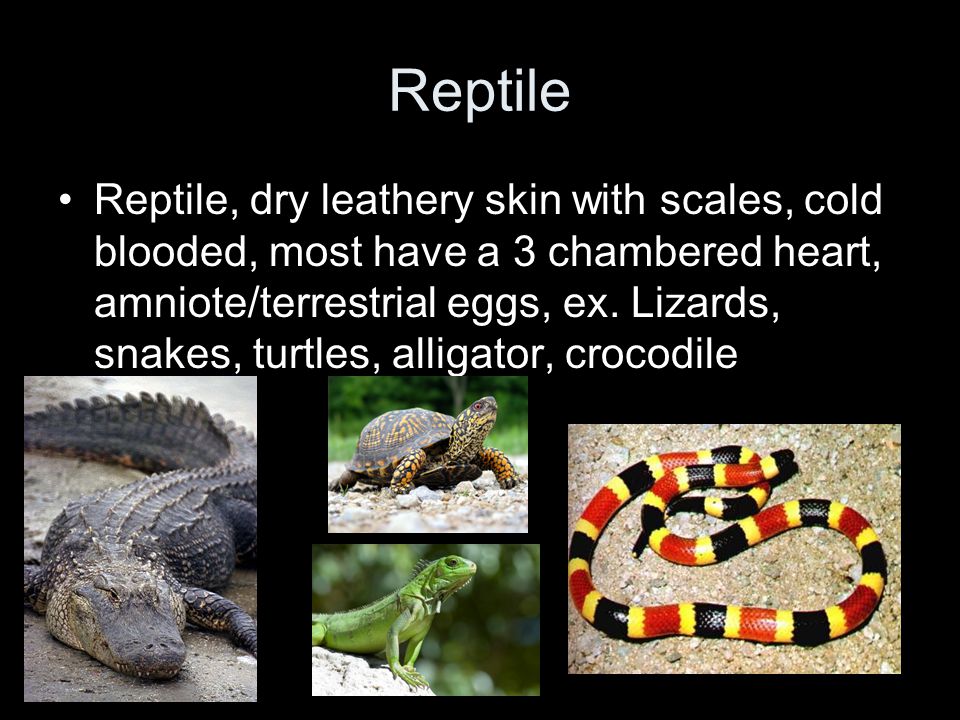The image appears to be an informational slide, likely from a PowerPoint presentation, detailing the characteristics of reptiles. At the top of the screen, a black rectangle contains white text emphasizing the term "Reptile," followed by a bullet-point list describing key traits: "Dry, leathery skin with scales," "Cold-blooded," "Most have a three-chambered heart," "Amniote," "Terrestrial eggs." Examples provided include lizards, snakes, turtles, alligators, and crocodiles. 

Beneath the text, four images are arrayed horizontally across the bottom of the screen. The bottom-left image depicts an alligator (mistaken for a crocodile in one description). Next, two centrally positioned images are stacked: the top image features a turtle (or tortoise), and the bottom image shows a lizard, likely an iguana. The rightmost image showcases a brightly colored snake lying in sediment. The color palette of the slide includes white, black, gray, brown, green, red, and yellow. The overall design is reminiscent of a PowerPoint presentation layout.